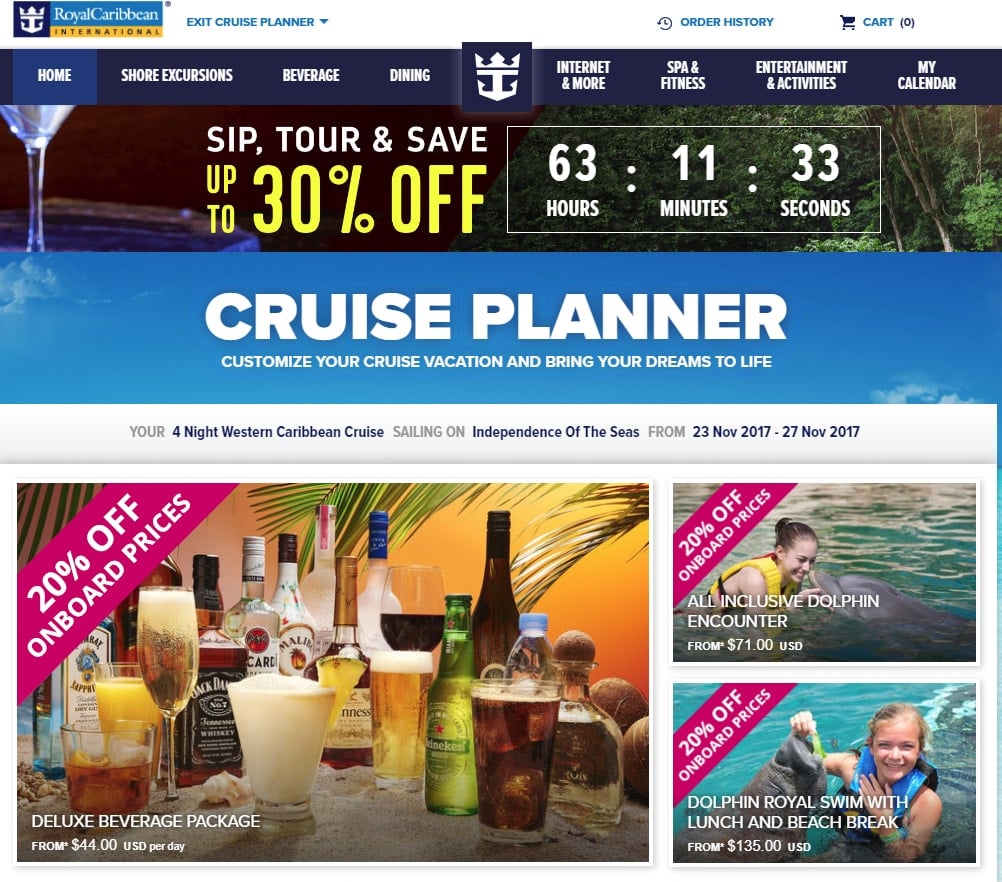This is a detailed caption for an image captured from the Royal Caribbean cruise planner page:

---

The image is a screenshot from the Royal Caribbean International's cruise planner webpage. In the top left corner, the Royal Caribbean International logo is prominently displayed beside the text "Exit Cruise Planner". Moving to the top right, there is an option labeled "Order History" next to an icon of an empty shopping cart. Below this section, a navigation border features various tabs including Home, Shore Excursions, Beverage, Dining, Internet and More, Spa and Wellness, Entertainment and Activities, and My Calendar, with the Home tab currently selected.

Directly below the navigation border, bold text reads "Sip, tour, and save up to 30% off" along with a countdown timer indicating 63 hours, 11 minutes, and 33 seconds remaining for the offer. Against a blue background, the text "Cruise Planner: Customize your cruise vacation and bring your dreams to life" is displayed prominently. Beneath this, detailed information about a four-night Western Caribbean cruise aboard the Independence of the Seas is provided, specifying the dates from November 23, 2017, to November 27, 2017.

The lower section of the image features promotional images and offers. On the left, there is an image showcasing various types of alcohol including Bacardi, Malibu, Jack Daniels, and Heineken, with palm tree fronds in the background and a banner that reads "20% off on-board prices". This is the Deluxe Beverage Package starting at $44 per day. Beside this image, on the right, there is another promotion showing "20% off on-board prices" for an "All Inclusive Dolphin Encounter" beginning at $71 USD. Below, a picture of a child with a dolphin accompanies the offer for "Dolphin Royal Swim with Lunch and Beach Break" priced from $135.

---

This detailed caption provides a comprehensive overview of the screenshot’s content, accurately reflecting the information presented on the Royal Caribbean cruise planner page.